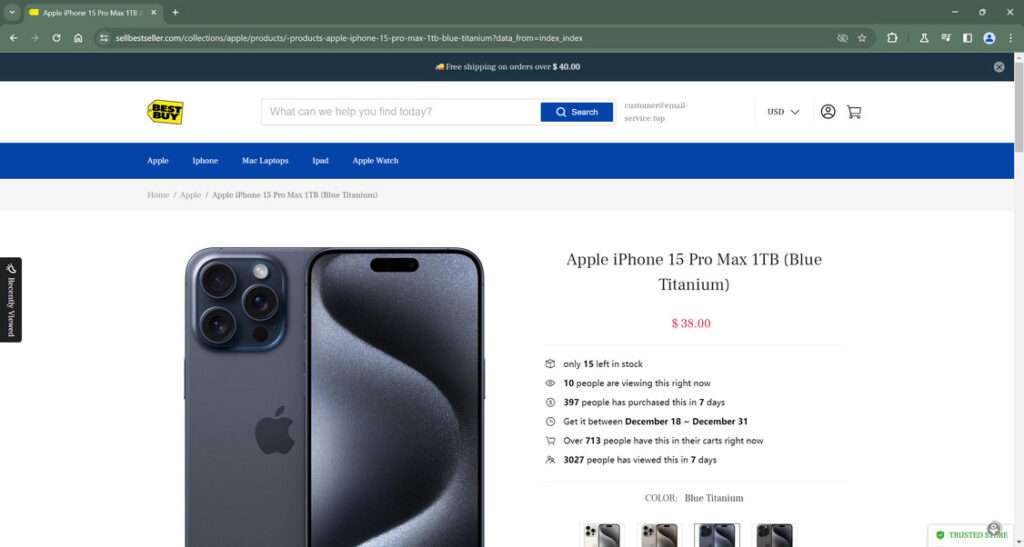**Screenshot Description: Best Buy Website Imitation Selling Apple iPhone 15 Pro Max 1TB in Blue Titanium**

This screenshot, most likely taken from a desktop browser, appears to be a forged version of the Best Buy website showcasing the Apple iPhone 15 Pro Max 1TB in Blue Titanium. The browser in use seems to be Google Chrome, evident from the layout and icons displayed.

### Browser Interface:
- **Top Left Corner:**
  - Browser tab displays "Apple iPhone 15 Pro Max 1TB" with the remaining text cut off.
  - A single tab is open.

- **Top Right Corner:**
  - Minimize (dash), maximize (stacked rectangles), and close (X) buttons, all appearing on a dark green background.

- **Navigation and Address Bar:**
  - Back arrow (left) and grayed-out forward arrow (right).
  - Refresh and home buttons, all in white.
  - Address bar contains a long, suspicious URL: `sellbestseller.com/collection/Apple/products-Apple-iPhone-15-Pro-Max-1TB-blue-titanium?data_from=index_index`.
  - An 'X' symbol possibly indicating privacy settings, an open star for bookmark (unselected), puzzle piece for extensions, flask icon, and several other extension icons described but not fully identified.
  - Three vertical dots on the far right corner for additional options.

### Website Interface:

- **Top Banner:** 
  - Dark blue banner stating: "Free shipping on orders over $40" in white text. To the left, a yellow icon is not fully visible, and a gray 'X' on the right to close the banner.
  
- **Logo and Search Bar:**
  - A questionable Best Buy logo (yellow price tag with "Best Buy" in bold letters).
  - Search bar with placeholder text: "What can we help you find today?" in gray.
  - Blue search button with a magnifying glass icon.
  - Additional two gray words to the right, partially illegible.
  - 'USD' dropdown for currency selection.
  - Person icon for account settings and a shopping cart icon.

- **Navigation Menu:**
  - A blue navigation menu with white text for categories: "Apple, iPhone, Mac, laptops, iPad, Apple Watch."
  - Below, breadcrumb navigation: Home > Apple > Apple iPhone 15 Pro Max 1TB (Blue Titanium).

### Product Page:

- **Product Display:**
  - Left side shows the back of the iPhone 15 Pro Max in blue titanium with a square module housing three camera lenses and the Apple logo.
  - Right side depicts the front of the phone with a wavy gray gradient wallpaper.

- **Product Description:**
  - Title: "Apple iPhone 15 Pro Max 1TB (Blue Titanium)."
  - Price: "$38.00" in red, which is suspiciously low for such a device.
  - Stock and Viewing Statistics:
    - "Only 15 left in stock" with the number 15 in bold.
    - "10 people are viewing this right now," with the number 10 bolded.
    - "397 people have purchased this in 7 days," and a clock icon.
    - "Get it between December 18 and December 31," with another clock icon.
    - "Over 713 people have this in their carts right now."
    - "3,027 people have viewed this in 7 days."

- **Product Options:**
  - Color selection displaying four options: white, beige, blue (selected), and black.
  - Bottom right includes a green shield icon labeled "Trusted Store."

### Additional Notes:
- Despite featuring the Best Buy logo, the website URL and product details strongly indicate it's a fraudulent site.
- The extremely low price and various statistical claims aim to create a false sense of urgency and encourage immediate purchases.

In summary, the screenshot shows a possible scam site imitating Best Buy, presenting a detailed but highly suspicious product page for the Apple iPhone 15 Pro Max 1TB in blue titanium.